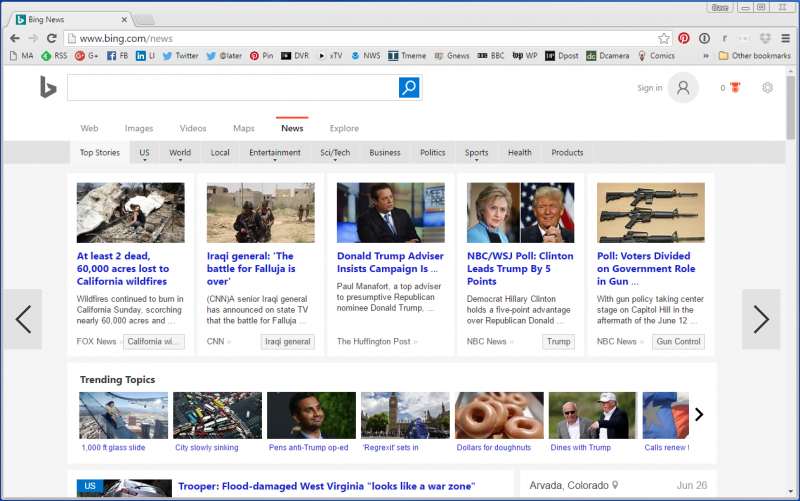**Detailed Caption for the Bing News Landing Page Image:**

This image captures a landing page from Bing News displayed in a web browser. The browser shows only one open tab, and the URL in the address bar is "www.bing.com/news". The page features five highlighted news stories, each accompanied by a relevant image.

1. **Headline 1**: "At Least Two Dead, 60,000 Acres Lost to California Wildfires" – This story highlights the devastating impact of wildfires in California, indicating significant loss of life and property.
2. **Headline 2**: "Iraqi General: The Battle for Fallujah is Over" – This article reports on a decisive moment in the conflict in Fallujah, Iraq, narrated by a military general.
3. **Headline 3**: "Donald Trump Advisor Insists Campaign is..." – The title trails off due to its length, suggesting additional details about the Trump campaign not fully visible.
4. **Headline 4**: "NBC/WSJ Poll: Clinton Leads Trump by Five Points" – This report presents polling data indicating a lead for Clinton over Trump.
5. **Headline 5**: "Poll: Voters Divided on Government Role in Gun..." – The incomplete headline implies a discussion around voter sentiments regarding government involvement in gun control.

Below these featured stories is a list of trending topics, each with a brief caption and associated image. These captions are:

1. "1,000 Foot Glass Slide"
2. "City Slowly Sinking"
3. "Paris Anti-Trump Op-Ed"
4. "Regrets It Sets In"
5. "Dollars for Donuts"
6. "Dines with Trump"
7. "Calls Renew..." – This title is also partially visible due to the horizontal scrolling format of the trending topics section.

The layout and representation of content suggest that the page is designed to offer a quick glance at significant news items and trending topics, keeping the reader updated on the latest events and opinions.